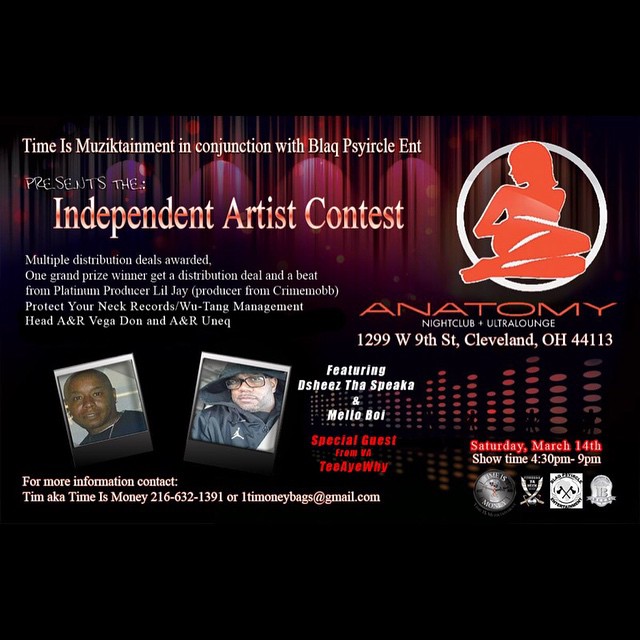This advertisement is for a special event at the Anatomie Nightclub, an ultra lounge located at 1299 West 9th Street, Cleveland, Ohio 44113. The central theme is the "Independent Artist Contest," presented by Time Is Music-tainment in conjunction with Black Circle Entertainment. 

The top half of the ad features a red and black curtain background, with bold white text detailing the event. On the left side, additional white text provides more information, while the lower left corner showcases two color photos of male artists. The right side highlights the red logo of a reclined woman inside a white circle, with the word "Anatomy" boldly written below it. 

This event promises multiple distribution deals for award-winning artists, with a grand prize including a beat from Platinum producer Lil J (known for his work with Crime Mob), and participation from Protect Ya Neck Records and Wu-Tang Management's head A&R, Vega Don, as well as Unique. Featured performers include "She Is The Speaker" and "Mellow Boy," with a special guest from B.A.T.I.

The event is scheduled for Saturday, March 14th, with showtime from 4:30 p.m. to 9:00 p.m. For more information, interested parties can contact Time (aka Time Is Money) at 216-632-3139 or via email at timoneybags@gmail.com.